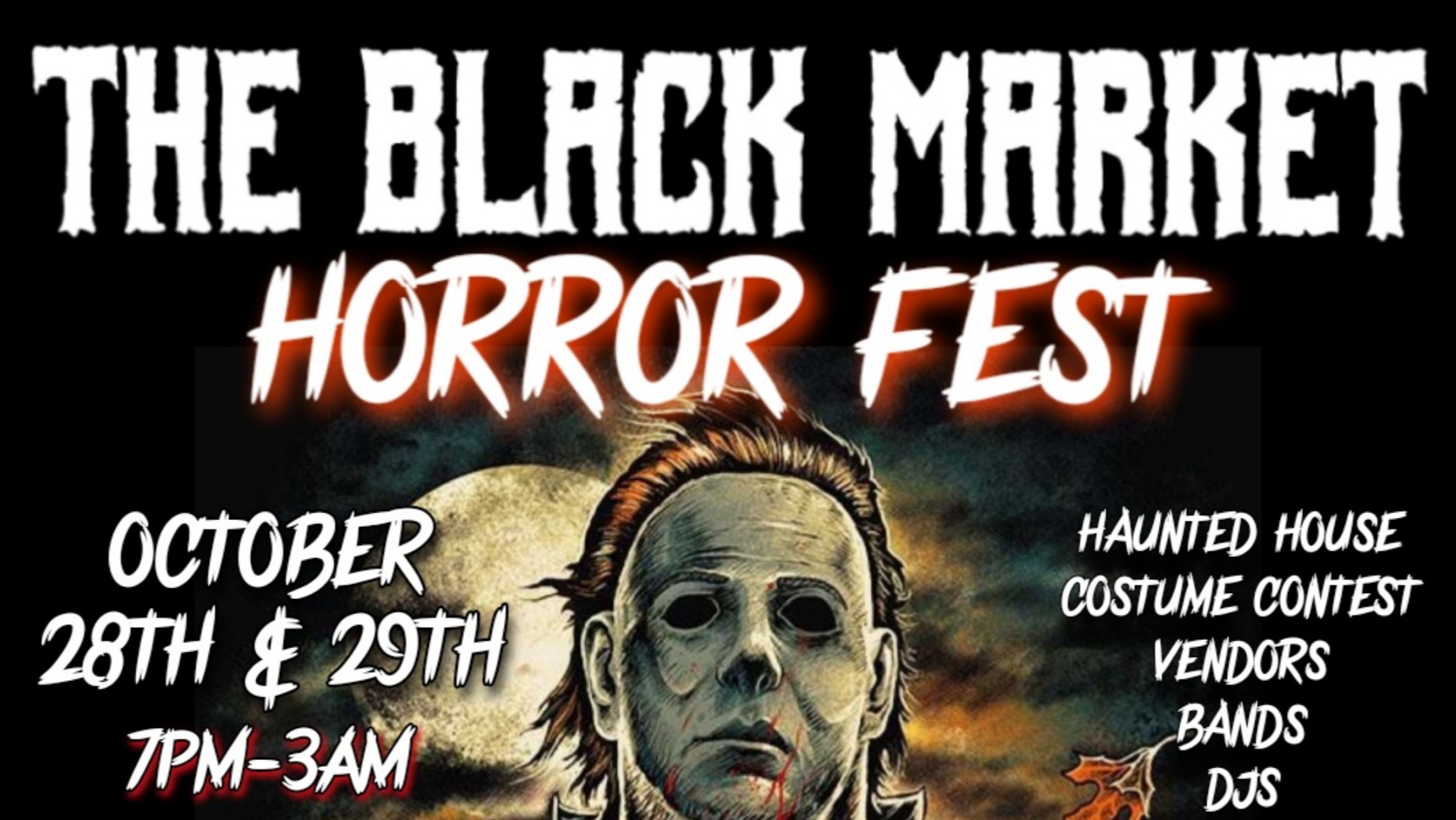This rectangular advertisement poster, wider than it is tall, features a chilling, dark design perfect for Halloween. The background is predominantly black with a lighter, eerie section in the middle suggesting a full moon with an orange and gray tint to the sky. At the top, in creepy white letters, the title "The Black Market" is displayed using a scary font. Beneath that, in the same spooky font but bordered in red, the text announces "Horror Fest." 

At the lower left, white letters detail the event timing: "October 28th and 29th, 7pm-3am," while the right side lists attractions in white text: "Haunted House, Costume Contest, Vendors, Bands, DJs." Dominating the center of the poster is the unsettling face of a monster, bearing a striking resemblance to Frankenstein. The figure features reddish hair, empty eye holes, and bolts in the neck, completing the spectral theme. The spooky backdrop highlights an ominous moon and falling autumn leaves, enhancing the eerie atmosphere of this Halloween event.